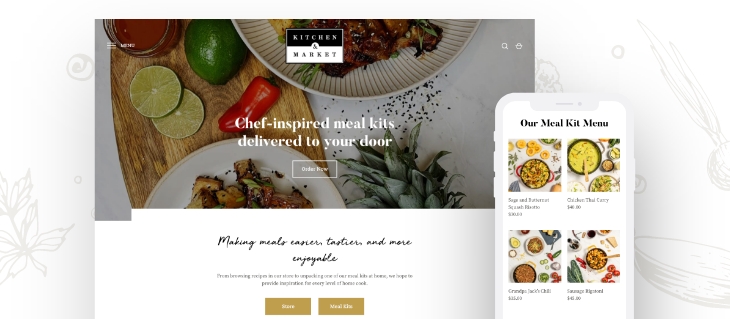The image depicts a screenshot showcasing the "Kitchen and Market" website as viewed on both a desktop computer (on the left) and a mobile phone (on the right). The website header features a clean and cohesive design with the brand's logo positioned prominently at the top. The "Kitchen" portion of the logo is set against a small black background, while the "Market" portion is against a white background. Directly beneath the logo, the tagline reads, "Chef Inspired Meal Kits Delivered to Your Door."

The desktop version provides a visually appealing header image featuring a rustic cutting board adorned with fresh ingredients: two lime slices, a whole lime, a red chili, and two plates with prepared meals—one positioned atop the board and the other to its side, all set on a white surface, exuding a clean and inviting appearance.

To the right, the mobile phone screen displays a streamlined version of the website with the header text "Our Meal Kit Menu" at the top. Below this header are four images corresponding to different meal kits, each accompanied by their respective names, descriptions, and prices. This layout suggests that "Kitchen and Market" is a food delivery service specializing in chef-prepared meal kits that are conveniently delivered to customers' doors.